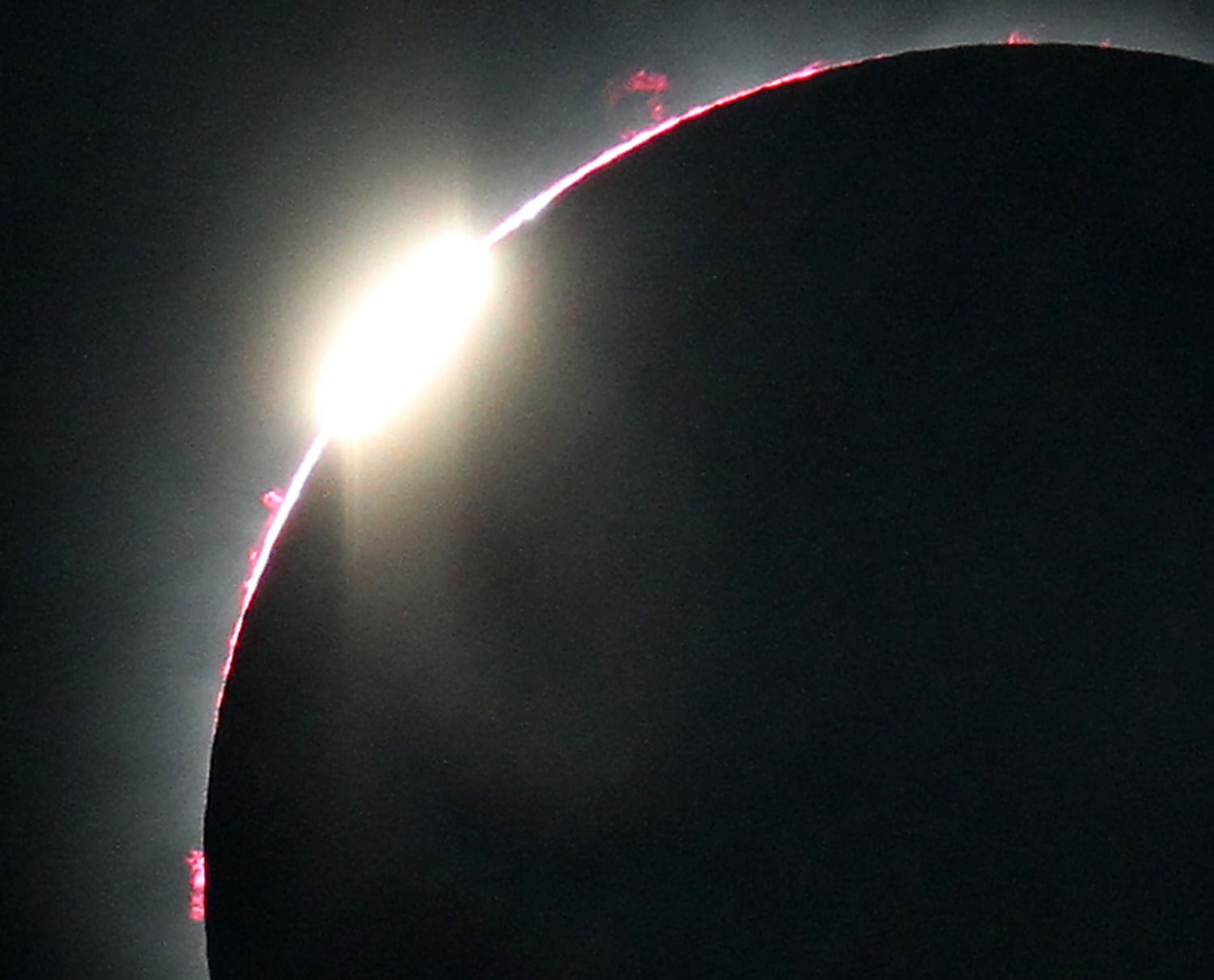This detailed close-up photograph captures a dramatic moment during a solar eclipse. The background is a deep, solid black, setting a stark contrast against the celestial event. Dominating the image, a dark circular shape, presumably the moon, spans from the top right to almost the bottom left, covering approximately three-quarters of the frame. The darkness envelops the entire right-hand side of the photo. Toward the upper left, sunlight brilliantly peeks through the moon's edge, creating a powerful burst of light known as the "diamond ring" effect. Surrounding this intense white light, a subtle but vivid pinkish-red hue appears along the edge of the moon, likely representing solar flares or prominences. Scattered along this edge are tiny pink or reddish spots, possibly stars or additional solar phenomena, adding to the captivating details of this astronomical event.